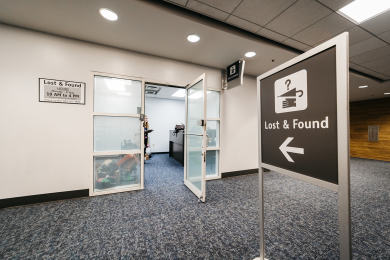The image depicts the interior of an office building, specifically focusing on the lobby leading to a 'Lost and Found' area. The floor is covered with a blue carpet, and the walls are trimmed with black rubber. Central to the room are two large metal-framed signs mounted on silver poles, featuring brown signage with white text that reads "Lost and Found" accompanied by arrows and a depiction of various lost items, including umbrellas and a question mark. These arrows point towards an open doorway with frosted glass doors and windows on each side. Through the glass doors, a room is visible with office furniture and a desk situated to the right, while a person stands on the left. To the left of this open doorway, a white sign with a black border repeats the "Lost and Found" text, affixed to a white wall. The suspended ceiling has built-in lights, contributing to a well-lit environment accentuated in shades of gray, white, brown, light brown, and tan.